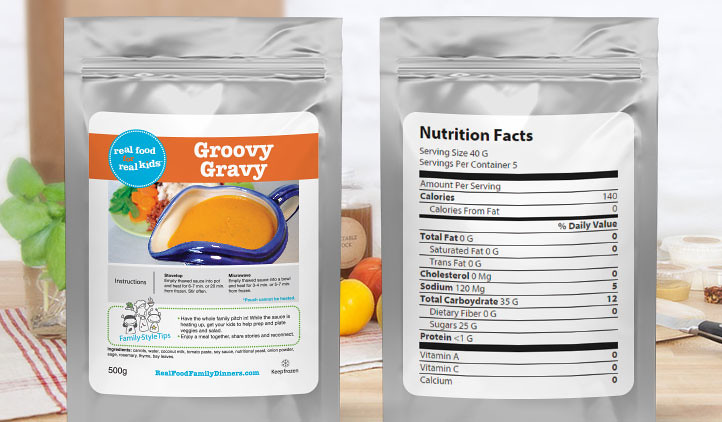The image features two silver-colored plastic packages of a product called "Groovy Gravy." The package on the left shows the front label, which includes an orange bar at the top with "Groovy Gravy" written in white. Above it is a blue circle with the text "Real Food for Real Kids" in white letters. Below this is an image of a blue-rimmed gravy boat filled with brown gravy. The background of the label depicts a green plate with vegetables such as parsley, sliced carrots, and possibly cauliflower or mashed potatoes. Additionally, instructional tips and family style tips are noted with too small text to read clearly. The bottom left corner of the label indicates the weight as 500 grams and the website "realfoodfamilydinners.com" written in red.

To the right of the first package is the back side of another identical package, featuring the nutrition facts in black text. It states the serving size as 40 grams, with 5 servings per container. Each serving contains 140 calories, 0 grams of total fat, 0 grams of saturated fat, 0 grams of trans fat, 0 milligrams of cholesterol, 120 milligrams of sodium, 35 grams of total carbohydrates (12% daily value), 0 grams of dietary fiber, 25 grams of sugars, and less than 1 gram of protein. It also specifies 0% daily value for Vitamin A, Vitamin C, and calcium. The packages are placed on a tan-colored table with a red checkered cloth, surrounded by miscellaneous objects including basil leaves, lemons, carrots, and possibly a jar or kettle.